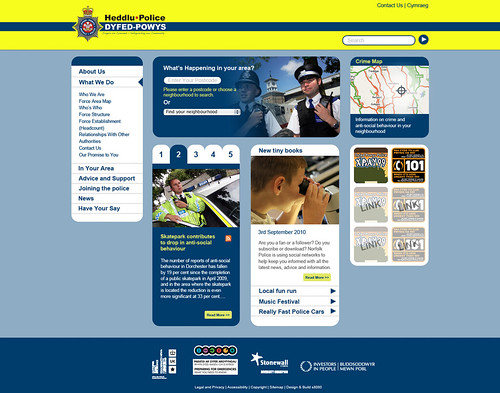**Website Front Page of Hadlu Police Department - Detailed Description**

The homepage of the Hadlu Police Department website features a structured and informative layout. At the very top, a horizontal yellow bar spans the width of the page, accented by a central blue stripe. On the left side of this bar, a detailed emblem is present. Although slightly obscured due to the zoom level, the logo appears to depict a crown atop a star, along with a grey rectangle, a red circle encircled by a blue ring, and additional symbols and text.

To the right of the emblem, bold text reads "Hadlu Police" followed by the letters "DYFED-POWYS." In the upper right corner of this section, the phrase "Contact Us" is clearly visible, accompanied by links for getting in touch with the department and a convenient search bar just below.

Beneath the yellow bar, the background transitions to a light blue area that contains various informational sections. On the right side, a prominent link directs users to the crime map. Adjacent to this on the left, a section titled "What's Happening in Your Area" invites visitors to enter their postcode to view local crime data. Additionally, a dropdown menu allows users to select their specific neighborhood.

To the left side of the main page, an organized menu lists several important links:
- About Us
- What We Do
- Who We Are
- Area Map for the Forces
- Contact
- In Your Area
- Advice and Support
- Joining the Police
- News
- Have Your Say

Further down the page, various clickable articles are available for in-depth reading. Moreover, links at the bottom showcase individuals and entities that support the Hadlu Police Department.